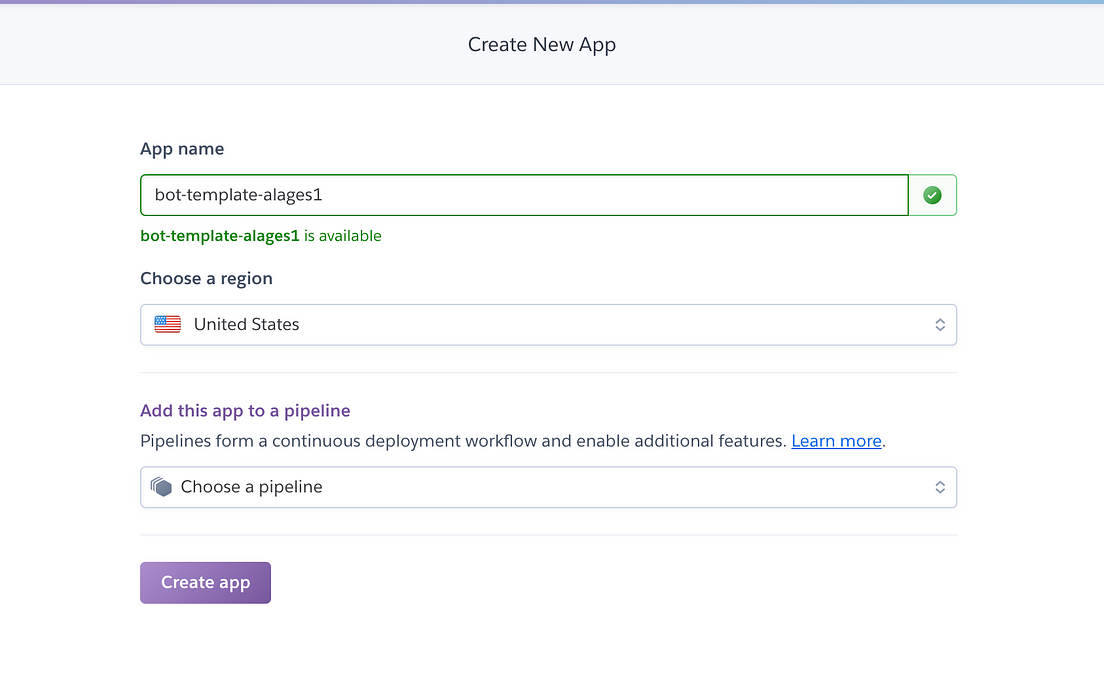The image depicts a user interface for creating a new application, likely in a web development platform.

At the very top, there is a thin, medium blue line, followed by a thin gray rectangular box. In black text within this gray box, it reads "Create a New App." Below this, the background is predominantly white.

The interface's first input section is for the app name. The designated input field currently contains the text "bot-template-alages1" and is highlighted with a green outline, indicating validity. A green checkmark beside the input confirms that "bot-template-alages1 is available."

Next, there is an option to choose a region, accompanied by a drop-down menu. The selected region is the United States, indicated by the United States flag on the left side of the drop-down.

Following this section, a thin gray horizontal line separates the subsequent elements. Below this line, in purple text, it reads "Add this app to a pipeline." Accompanying this text is an explanatory note stating, "Pipelines form a continuous deployment workflow and enable additional features." A blue hyperlink follows, offering users an option to "Learn more."

Another drop-down menu appears next, labeled "Choose a pipeline," accompanied by a small gray hexagon icon.

At the bottom left-hand corner of the interface, a purple button labeled "Create App" is prominently placed, guiding users toward finalizing the application creation process.